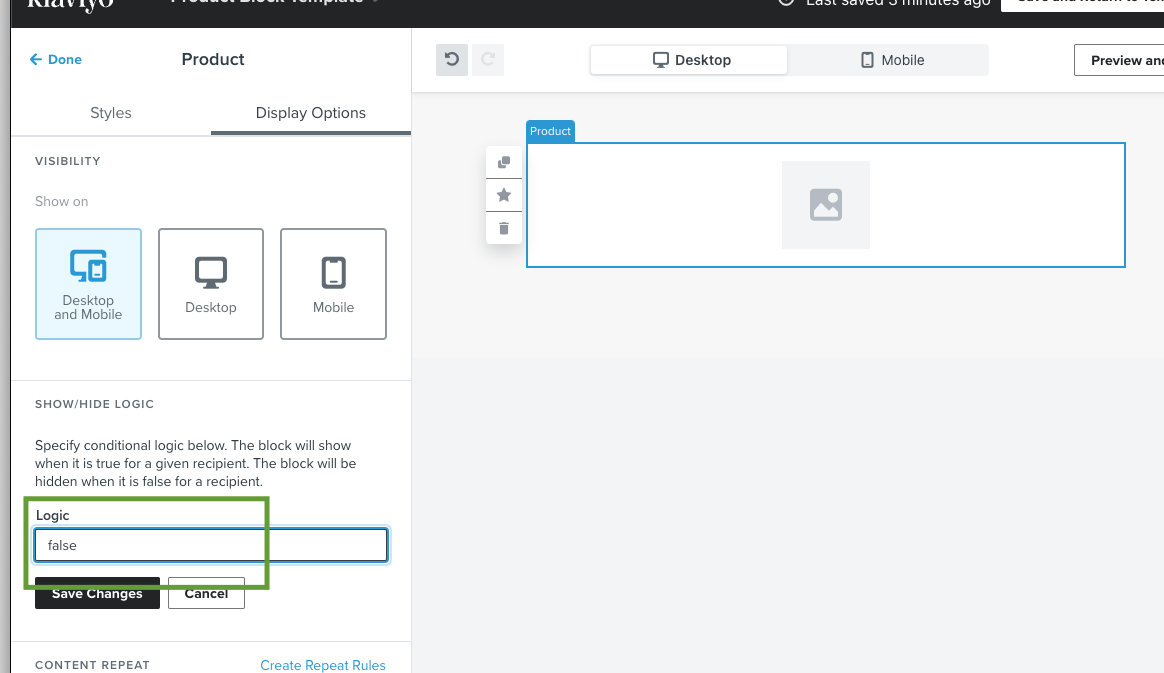This screenshot captures a detailed view of a website's interface on a desktop or laptop, featuring a comprehensive layout for configuring product display settings. At the very top, a partially visible black bar suggests the current status with a faintly legible phrase indicating "last saved five minutes ago." 

On the left side, a prominent white rectangular box labeled "Product" is highlighted in blue, accompanied by a left-pointing arrow and the word "Done." Beneath this, two selectable options are displayed: "Styles" and "Display Options," with the latter being active. 

The "Display Options" section offers visibility settings, with three checkboxes labeled for different devices: "Desktop and Mobile," "Desktop," and "Mobile." The "Desktop and Mobile" option is currently selected. Below this, a section titled "Show/Hide Logic" provides instructions to specify conditional logic, indicating that the block will be shown when true for a given recipient and hidden when false. 

A blue rectangular bar marked "False" is present, overlain by a slightly larger green bar labeled "Logic." Further down, there are "Save Changes" and "Cancel" buttons, followed by "Content Repeat" and an option to "Create Repeat Rules." The right-hand side is reserved for placing the product details.